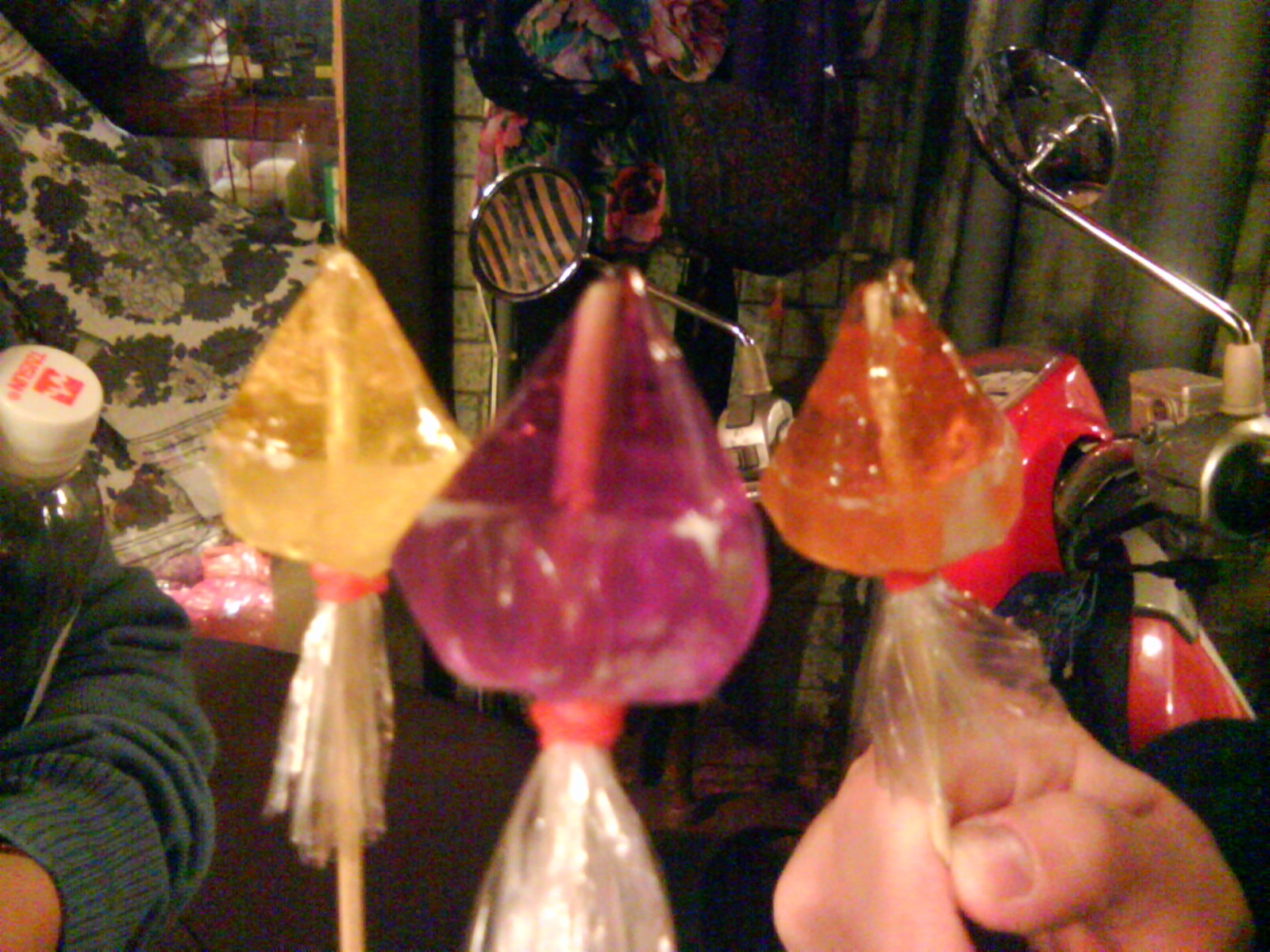In the foreground of the grainy photograph, a child's hand is seen holding one of three vividly colored lollipops, encased in clear cellophane with red tape securing them. The lollipops are brightly colored in orange, purple, and yellow hues, reminiscent of toy tops, each with a white stick inserted through them. The orange lollipop is gripped by the child's hand on the right side of the image. To the left, an adult arm in a blue or green sweater holds a bottle with a white cap that features red writing, obscured by the arm. In the background, which is dimly lit, there is a red motorbike or scooter with two round mirrors, positioned against a backdrop of green, white, and possibly floral-patterned curtains or wall hangings. A hint of hanging fabric adds a cozy clutter to the scene.